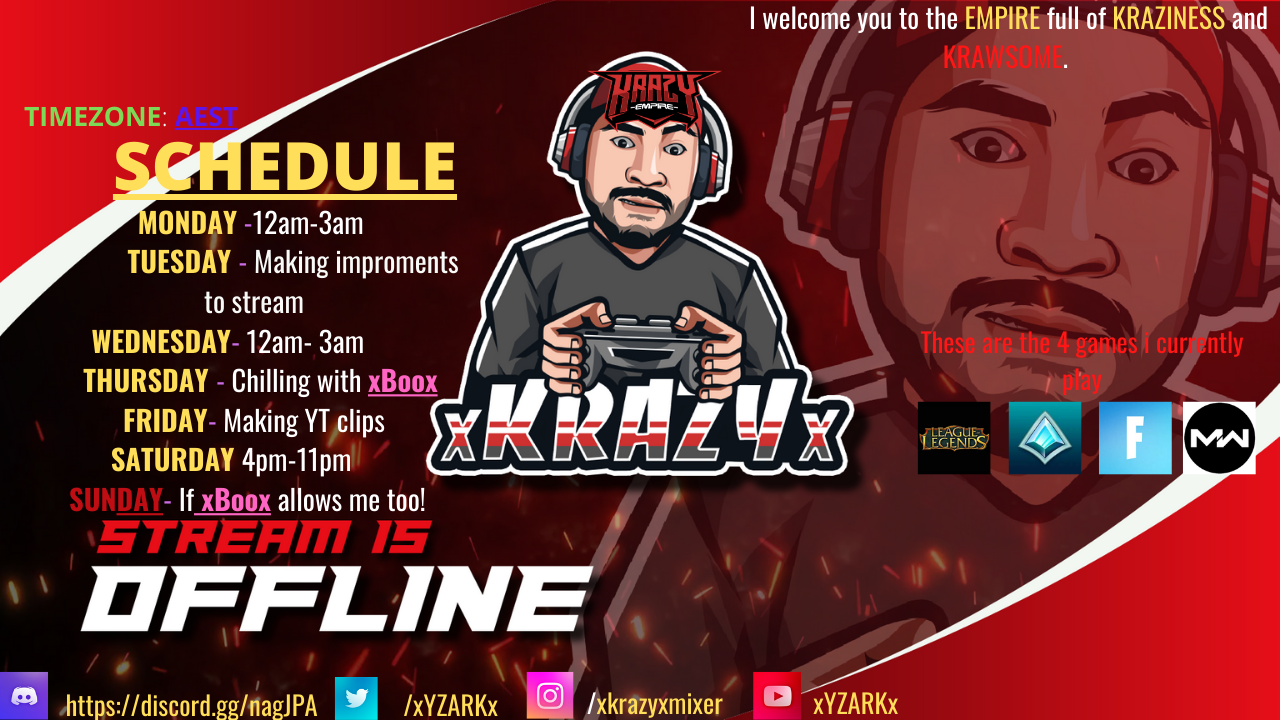This vibrant poster with a red background gradient from light to dark, primarily in the top left and bottom right corners, features a detailed graphic centered around a cartoon man with a mustache, wearing headphones and a black shirt with red accents. The man is prominently holding a black video game controller. Below him, bold text reads "X CRAZY KRAZY X" in an eye-catching mix of black, white, and red colors. The top right contains a welcoming phrase, "I welcome you to the empire full of craziness and cross them."

Adjacent to the left side of the poster, the man's gaming schedule is displayed in a variety of colors—yellow, white, hot pink, red, and green—designating his stream times in the AEST time zone:
- **Monday:** Midnight to 3 a.m.
- **Tuesday:** Impromptu streams
- **Wednesday:** 12 a.m. to 3 a.m.
- **Thursday:** Chilling with "XbooX" (likely a playful term for Xbox)
- **Friday:** Making YouTube clips
- **Saturday:** 4 p.m. to 11 p.m.
- **Sunday:** "STREAM is OFFLINE" if Xbox allows (noted in striking red and white font).

On the top right, beside the schedule, it lists the four games he currently plays, starting with "League of Legends" followed by three other game logos. The bottom left corner provides his social media handles with corresponding icons for Discord, Twitter, Instagram, and YouTube: 
- **Discord:** https://discord.gg/nagIPA
- **Twitter:** X Y Z A R K X
- **Instagram:** X crazy mixer
- **YouTube:** X Y Z R Z A R K X

Overall, the poster is a vibrant, dynamic, and detailed portrayal of a gamer’s streaming schedule and social media presence, all centralized around the engaging image of the gamer himself.